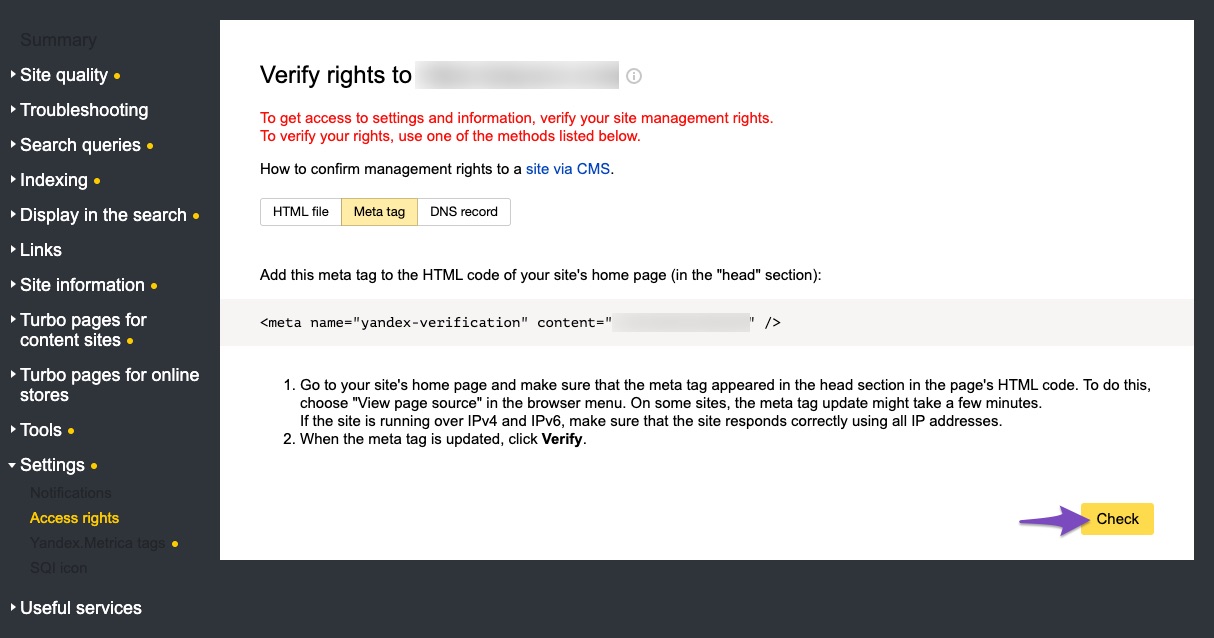The image displays a web interface with a detailed sidebar on the left. The sidebar contains a comprehensive list of options including: Site Quality, Troubleshooting, Search Queries, Indexing, Display in Search, Links, Site Information, Turbo Pages for Content Sites, Turbo Pages for Online Stores, Tools, Settings, Notifications, Access Rights, The Index, MedCert Tags, SQI Icon, and Useful Services. 

To the right of the sidebar, there is a large white box with a blurred title indicating "verify rights to" and a red instruction underneath that reads: "To get access to settings and information, verify your site management rights. To verify your rights, use one of the methods listed below." The methods mentioned for confirming management rights to a site include CMS, with an instructional note that follows. 

Below this, there are three buttons: a white button labeled "HTML File," a yellow button labeled "Meta Tag," and another white button labeled "DNS Record." Further down, there are instructions stating: "Add this meta tag to the HTML code of your site's home page in the head section." The meta tag to be added is styled as follows: `<meta name="yandex-verification" content=""/>`.